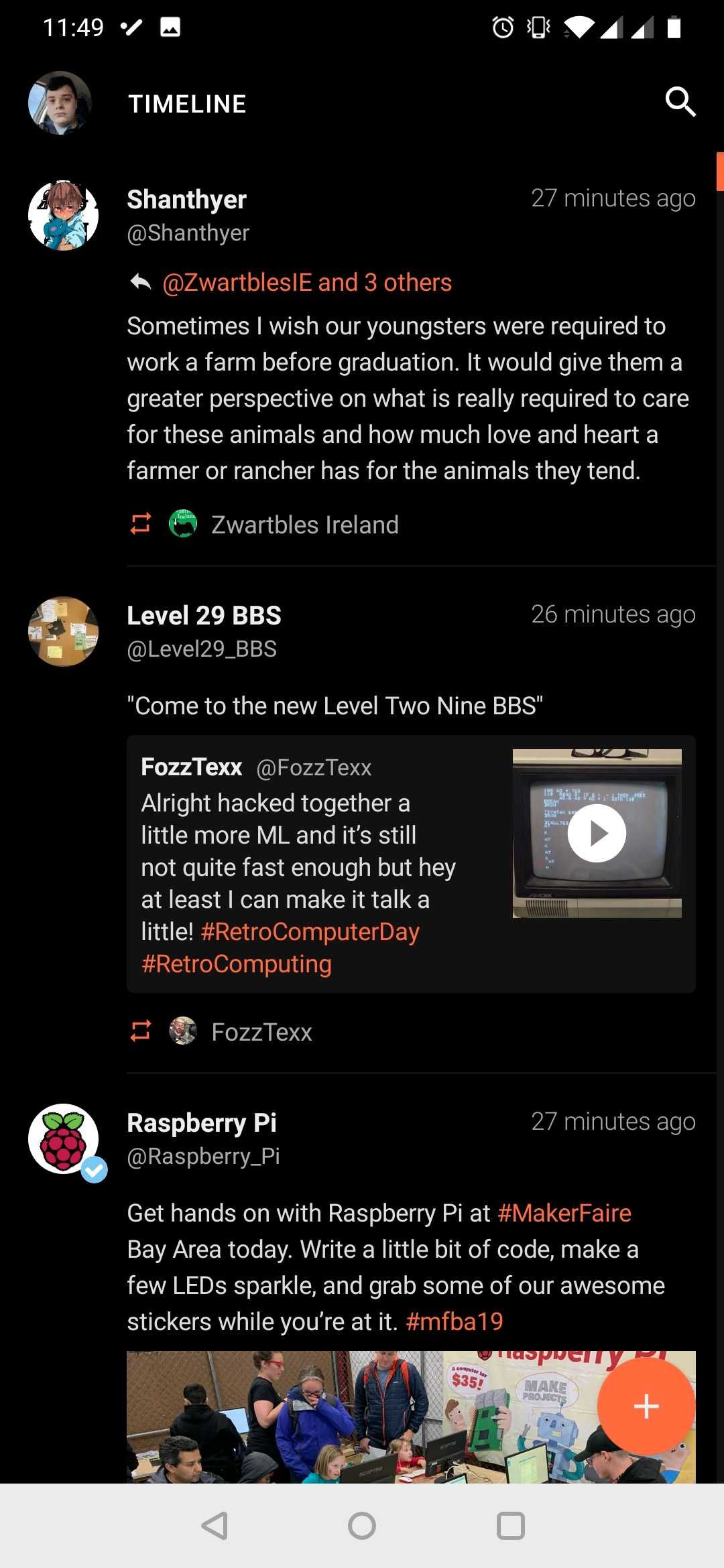This screenshot captures a detailed view of a Samsung smartphone's screen, displaying various notifications, icons, and a social media feed. It is 11:49 AM, as shown by the clock at the top. The status bar also indicates that the phone's alarm is set, the device is connected to WiFi, LTE is enabled, and the battery is nearly or completely charged.

The user's social media feed is visible, starting with a profile logo featuring someone sitting and looking down at the camera, likely taken inside a car. "Timeline" is displayed prominently in bold white letters, accompanied by a magnifying glass search icon on the right side.

Several comments populate the feed. The first comment, posted 27 minutes ago by user "shanthyer," expresses a nostalgic wish for youngsters to experience farm work before graduating, to understand the care and love farmers have for their animals. Following this is the label "swortables Ireland" and a red shuffle icon beneath each comment, along with a related green logo.

Another comment, which includes a video, was posted 26 minutes ago by "level 29 bbs." It discusses a project involving machine learning, mentioning that although the system isn't fast, it can now produce speech. This post includes hashtags like #retrocomputing and #retrocomputerday, and an invitation to "come to new level 29 bbs," with emphasized capital letters.

The final comment from "raspberry pi" mentions an event at Maker Faire Bay Area, encouraging attendees to engage with Raspberry Pi's booth, code LEDs, and grab some stickers. It includes the hashtag #mfba19. An orange circle with a white plus sign is positioned at the bottom right of the screen, likely an add or compose button.